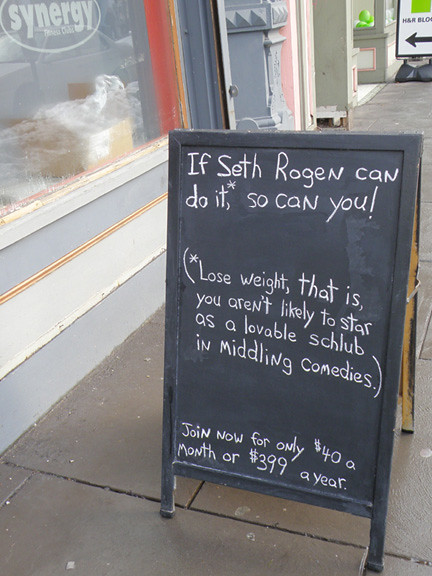The photograph captures a wet sidewalk, likely post-rainfall, in front of an older-style city block lined with turn-of-the-century storefronts. Prominently placed on the brownish-gray concrete sidewalk is a black sandwich board sign featuring a chalkboard panel. The sign reads in white chalk, "If Seth Rogen can do it, so can you!" and an asterisk leads to the clarification below: "Lose weight, that is. You aren't likely to star as a lovable schlub in middling comedies." Additionally, it advertises a membership deal: "Join now for only $40 a month or $3.99 a year." 

Behind the sign is a storefront with an orange-trimmed, large picture window displaying the words "Synergy," partially obscured by messy piles of cardboard boxes and plastic wrap. The building's façade is constructed of older wood. Adjacent shops similar in style can also be seen lining the sidewalk. In the distance, another sign with an arrow points towards H&R Block, indicating its location nearby.